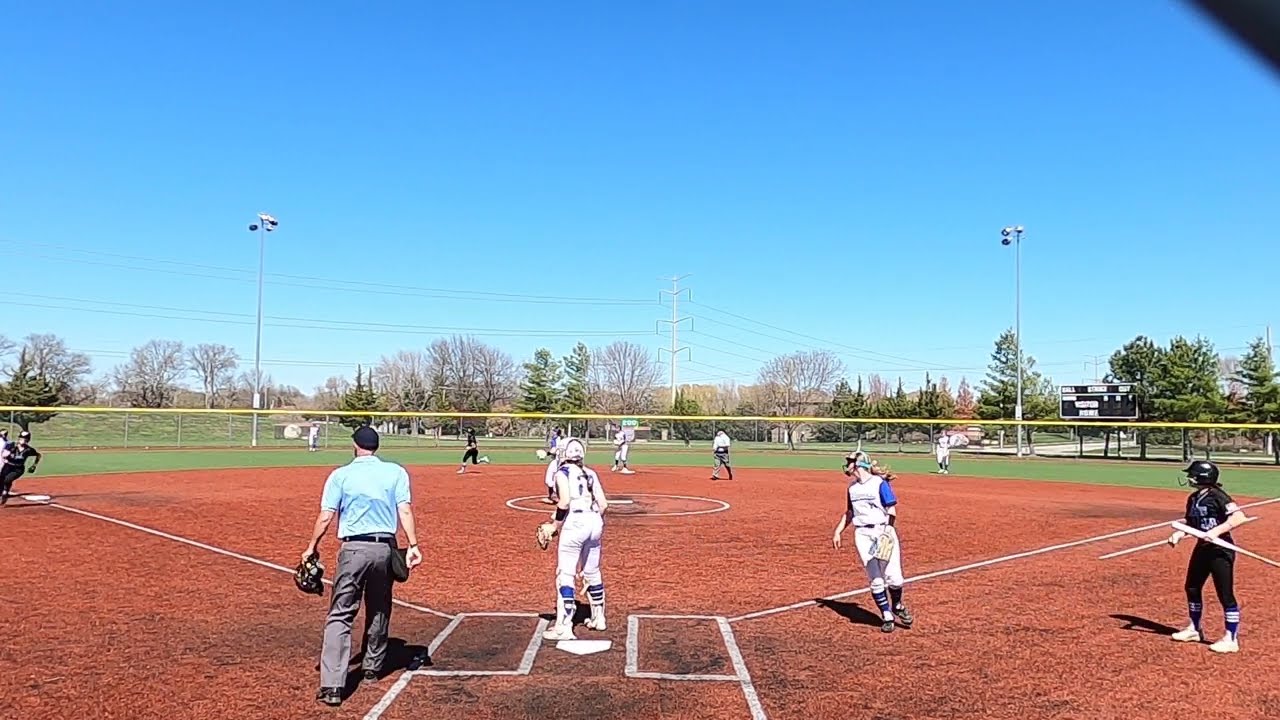This vibrant outdoor scene captures an intense moment in a women's baseball or softball game, viewed from behind home plate. The diamond, made of reddish-brown clay, is surrounded by lush green grass and bounded by a fence with a distinct white top. Under a clear, cloudless midday sky, two light posts stand guard in the background, amidst trees and power lines, with distant hills adding to the picturesque setting.

On the field, the team in black uniforms is up to bat, while the team in white uniforms with blue trim mans the outfield. A poised catcher, likely preparing for a critical tag, stands at home plate as runners are in motion—one darting from second to third and another sprinting from third towards home. Behind the catcher, an umpire clad in a blue shirt and gray trousers closely observes the play. A black scoreboard with white letters is faintly visible in the distance, though the score remains indistinguishable.